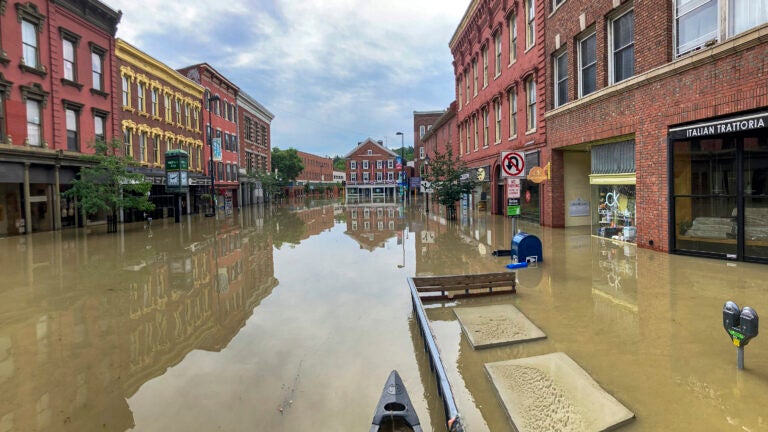This is a detailed photograph of a flooded street in a town or city. The street is completely submerged under brown, muddy water, reaching halfway up a blue mailbox, and nearly covering parking meters, signboards, and street lights. Both sides of the street are lined with old-fashioned red brick buildings adorned with numerous windows. In the background, a house with a triangular roof is visible. Amidst the submerged items, we also see a canoe, indicating that locals may be using it for transportation. Tall trees are scattered along the sides of the street, and the entire scene is captured under a blue sky dotted with white clouds. The reflection of the buildings and the sky on the water’s surface further emphasizes the extent of the flooding.